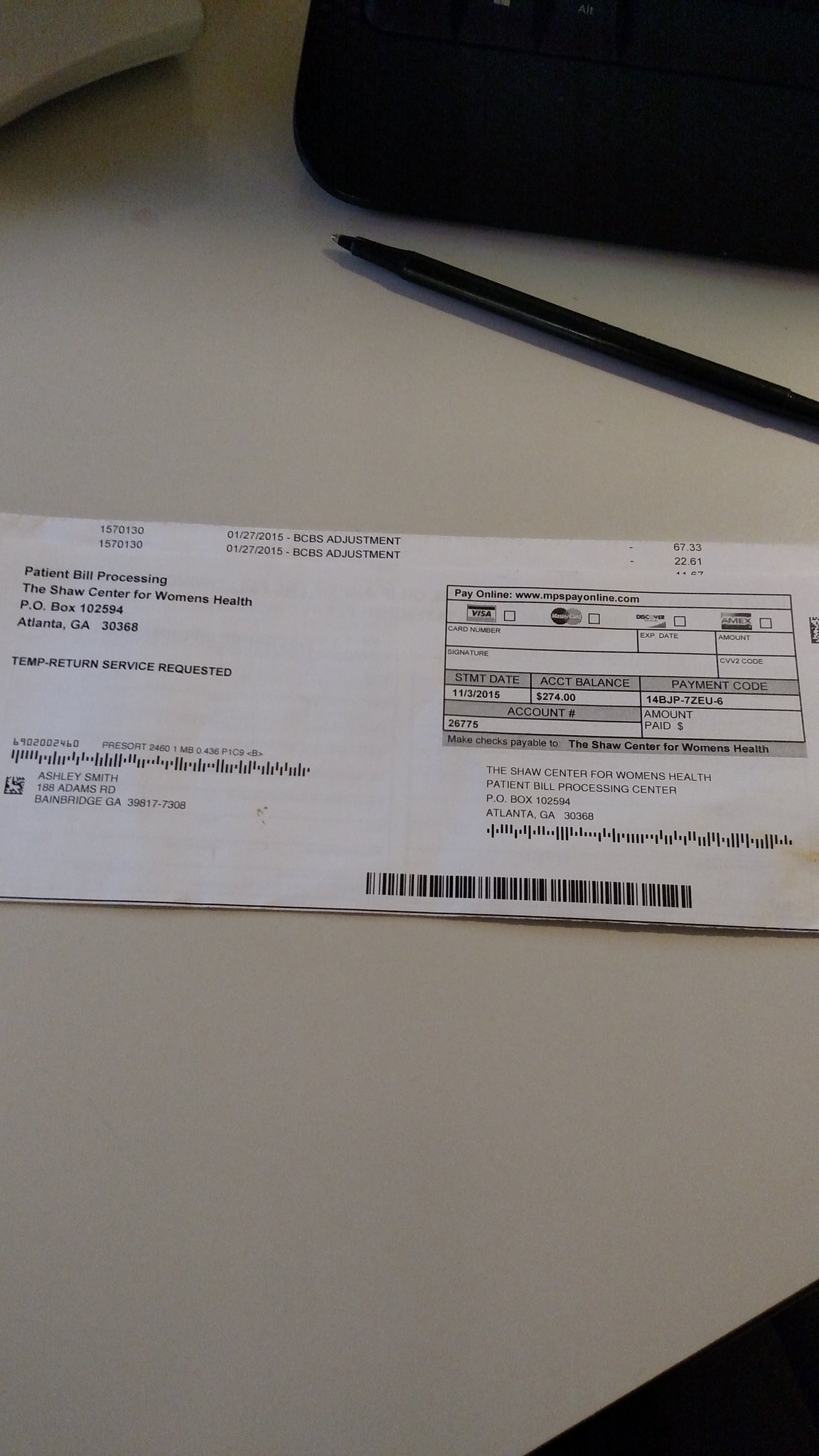The photograph captures a medical bill from the Shaw Center for Women's Health, based in Atlanta, Georgia, addressed to Ashley Smith. The bill is placed diagonally on a light-colored cream or white desk. Resting just above the bill is an uncapped black ballpoint pen. A black item with a curved corner, likely a computer keyboard, is partially visible above the pen. The bill, which reportedly dates to November 3, 2015, details patient bill processing and has an account balance of $274. There are several boxes on the right side of the bill for different payment methods. The presence of additional small white objects in the left-hand top corner adds to the clutter on the desk.